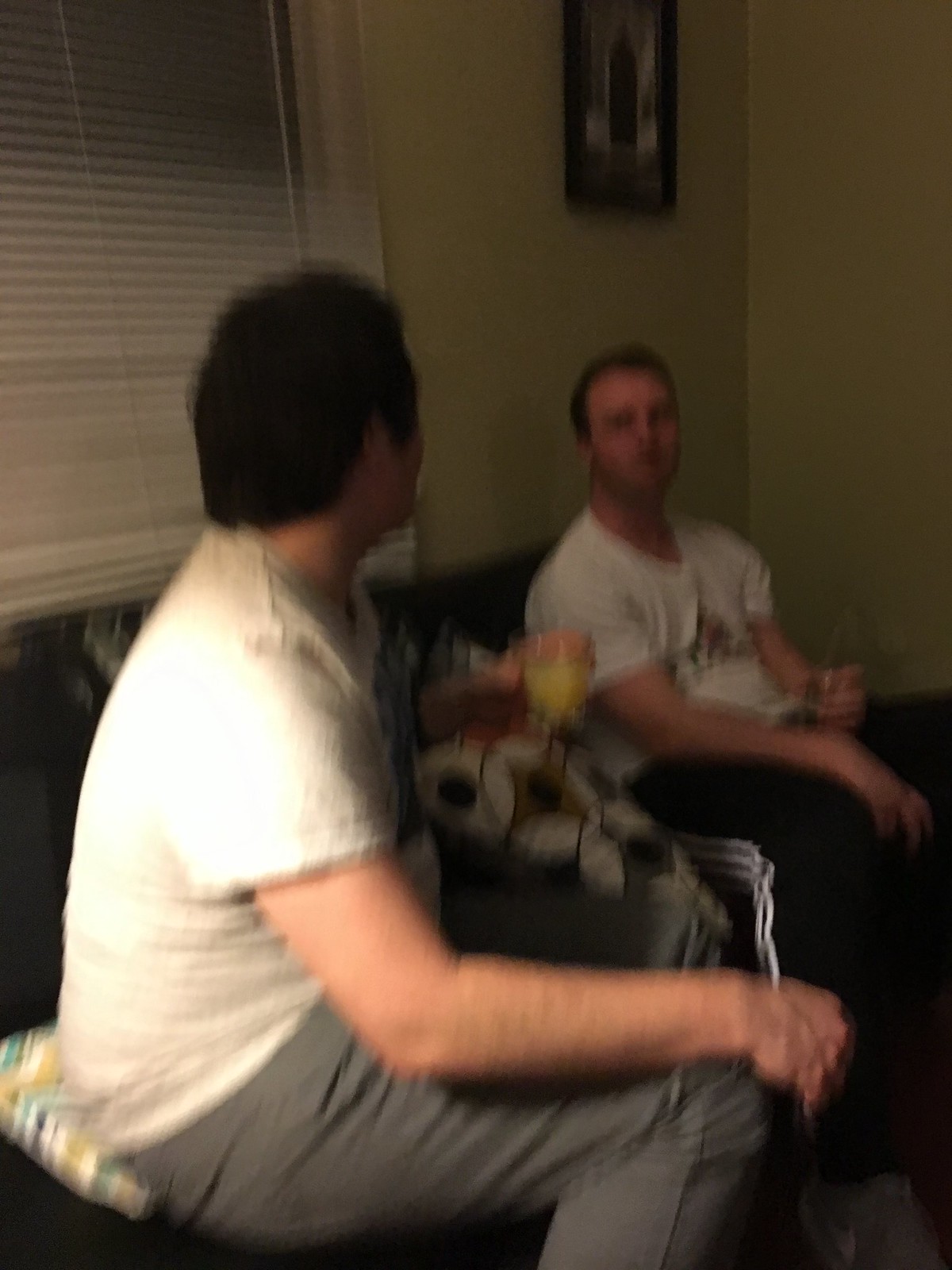In this portrait-oriented, slightly blurry photograph, two younger men, likely in their 20s, are sitting on opposite ends of a black couch in a dimly lit room. Both are wearing white t-shirts and different types of pants; the man in the foreground has on grey pants, while the other sports black tracksuit pants with white stripes down the side. 

The man in the foreground, who has short black hair, is turned sideways with his right forearm resting on his thigh and his left arm leaning on a patterned cushion that includes black, white, grey, and yellow geometric designs. He holds a glass of yellowish juice in his left hand as he engages in conversation with the other man. This second individual, with short dark brown hair, is facing the camera more directly but remains quite blurred. He also holds a glass, though the liquid inside is indiscernible. 

Behind them, the room features a yellow plaster wall, a window with horizontal white blinds pulled down, and a framed painting that appears to depict a building with a dark doorway. The overall scene conveys a cozy yet slightly obscure atmosphere.